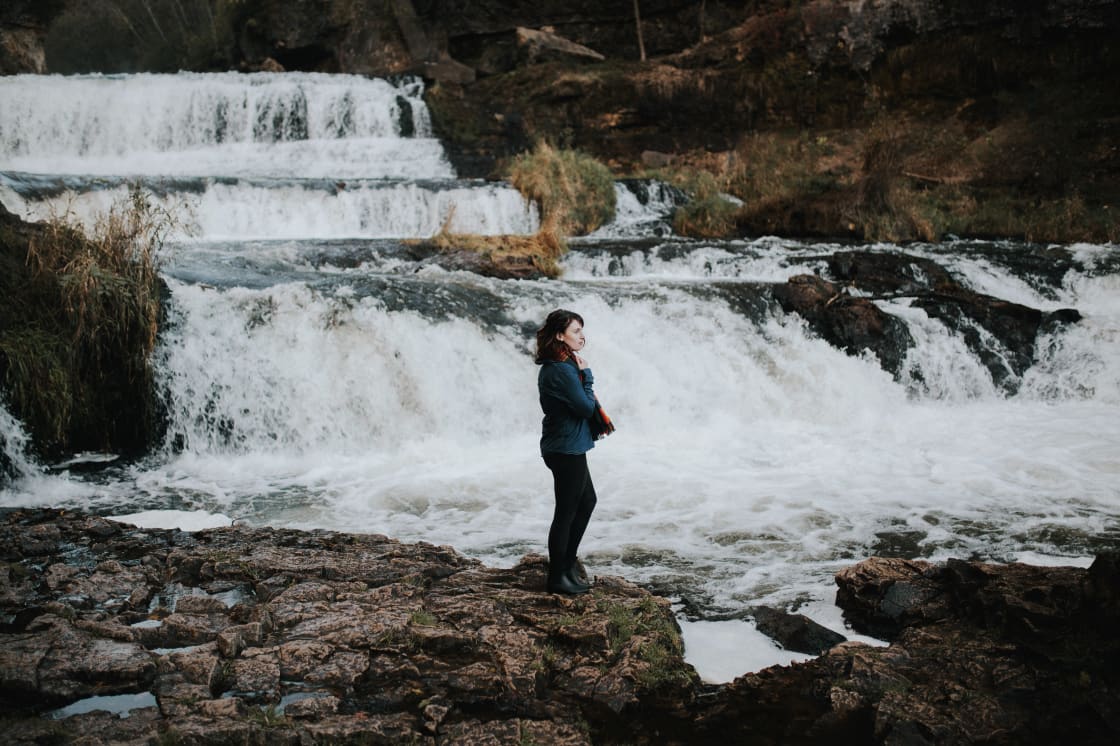In this high-resolution photograph taken in a natural setting, a woman stands on moss-covered brown rocks with a series of cascading waterfalls behind her. The water, rushing down multiple levels of rocky terrain, is turbulent and white, suggesting quick movement and rapids. The scene is enveloped in a dim, potentially sunset lighting, adding a dramatic touch. The environment appears cold, with dry and sparse vegetation visible on the hillside in the background. The woman, who has fair skin and long dark hair, is dressed in black pants, black shoes, and a long-sleeve blue top. A red and blue scarf is wrapped around her neck. She stands with one knee slightly bent, looking off to her right at something outside the frame, adding an air of contemplation to the serene yet powerful natural landscape.